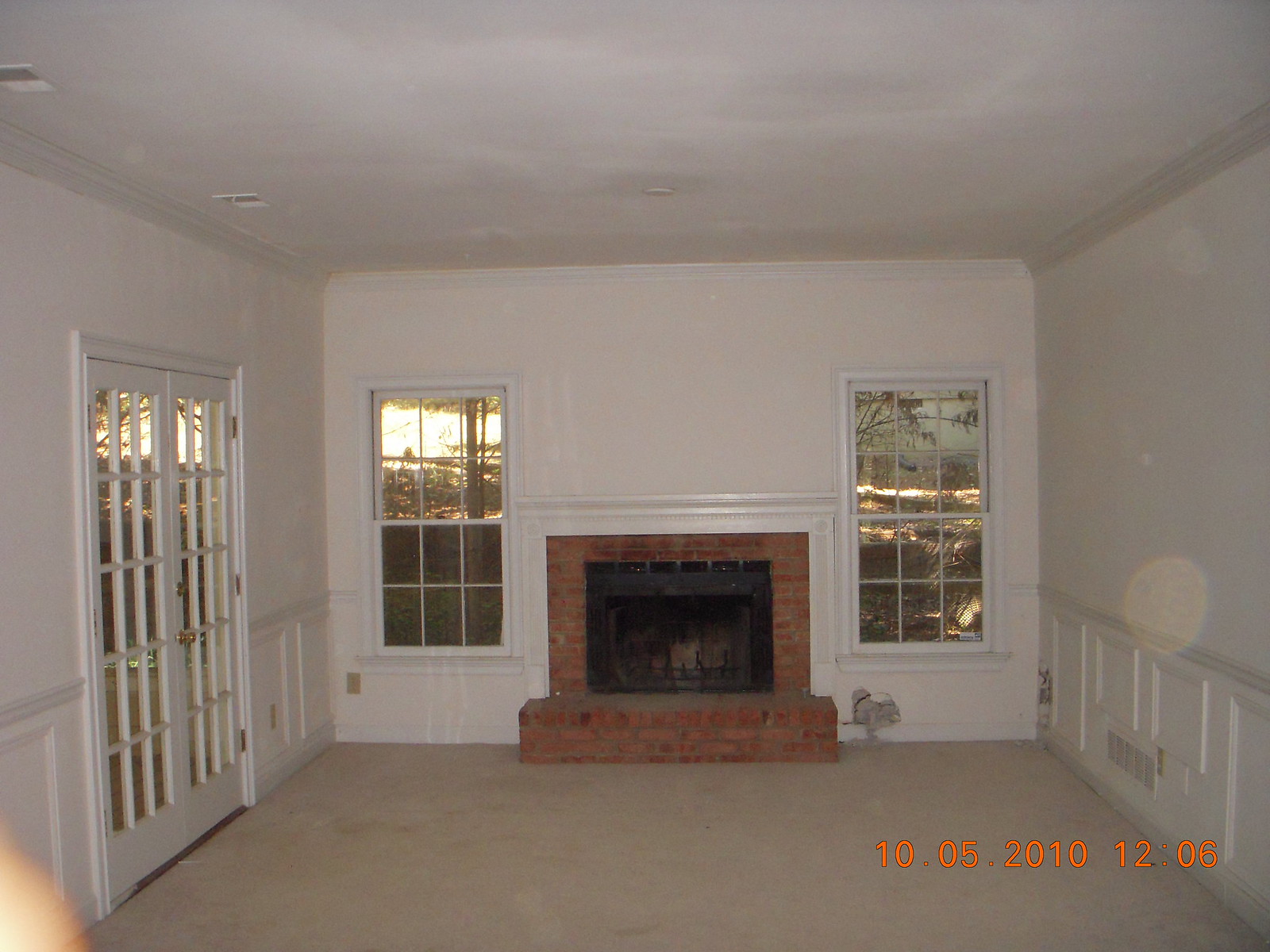The photograph captures a detailed view of a room interior. The central focal point is a red brick fireplace, styled from the 70s, which extends to about half the ceiling height and features a black grate and trim. Below it, there's a matching brick stoop. Flanking the fireplace are two large windows, framed in white wood, allowing an ample view of an outdoor scene, likely during sunset, as the lighting suggests.

The walls of the room are off-white and feature a wood border or chair railing, running partially up the walls. The right wall, like the others, is off-white and has a bottom border with engraved wood detailing. There's a small gray fan on the floor below the right window, and a couple of air vents can be seen on the ceiling's left side.

On the left wall, quarter-way up, there's the same wooden border, and two French doors with multiple small window panes open up to a yard. These doors are trimmed similarly in white wood. The flooring is a beige carpet, adding warmth to the room.

In the bottom left corner of the photograph is a shadow, possibly from the photographer's finger, while the bottom right corner has an orange timestamp reading "10-05-2010 12:06," indicating the date and time the photo was taken.